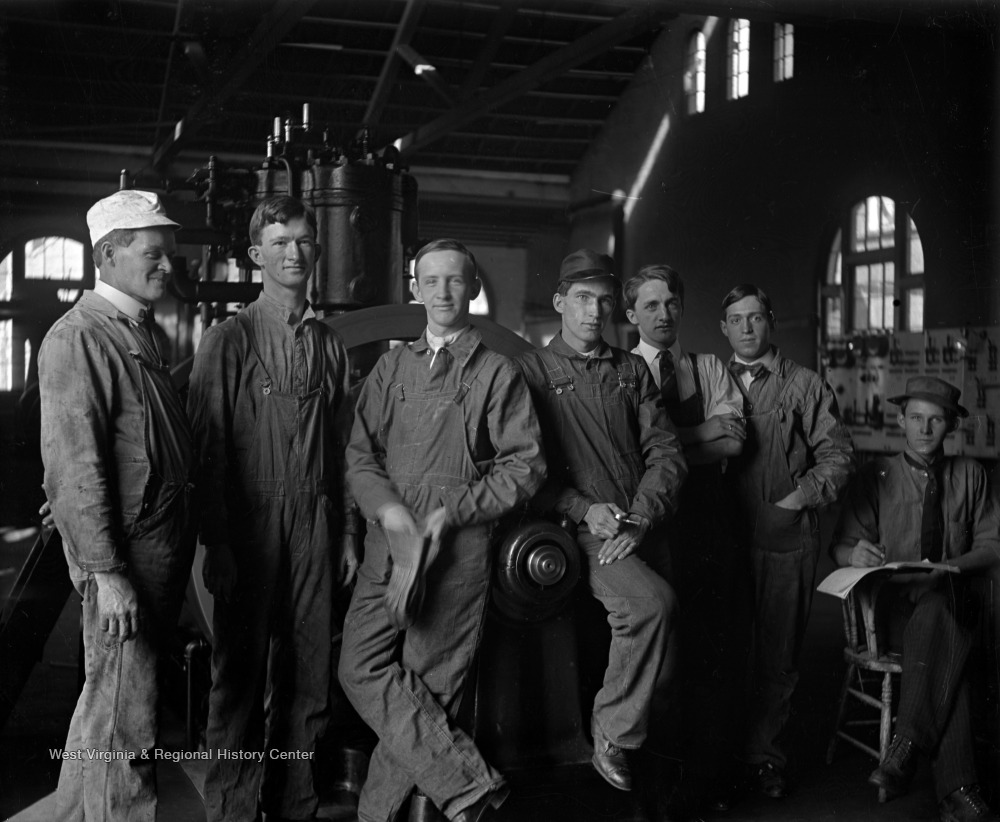This black and white vintage photograph, bearing the inscription "West Virginia and Regional History Center" in the lower-left corner, features seven men posing in an industrial factory or machine shop, likely from the 1930s or 1940s. The backdrop reveals high, trussed ceilings with peaked windows, and an assortment of machinery, including a noticeable steam engine that hints at a power-generating station.

The men, all white, are dressed in a mix of work attire, prominently featuring overalls and coveralls. At the far right, a man sits in a wooden chair, writing in a notebook, dressed in a dark shirt, black tie, and hat. Next to him, a younger man sports a white collared shirt paired with a bow tie under his overalls. The man in the center stands out with his white shirt and full black apron, also accompanied by a regular tie. To his right, another man is dressed in a white collared shirt and formal shoes under his coveralls. Further left, a younger man with a slicked hairstyle and a bow tie complements his coverall attire.

The leftmost man smiles, wearing a white hat over his coveralls, with a collared shirt peeking underneath. The remaining men are similarly clad in workwear, with some variations in their shirts and accessories. The ambiance of the photo, with visible machinery and detailed structural elements, captures a moment in a historical industrial setting, reflecting the era's work culture and attire.